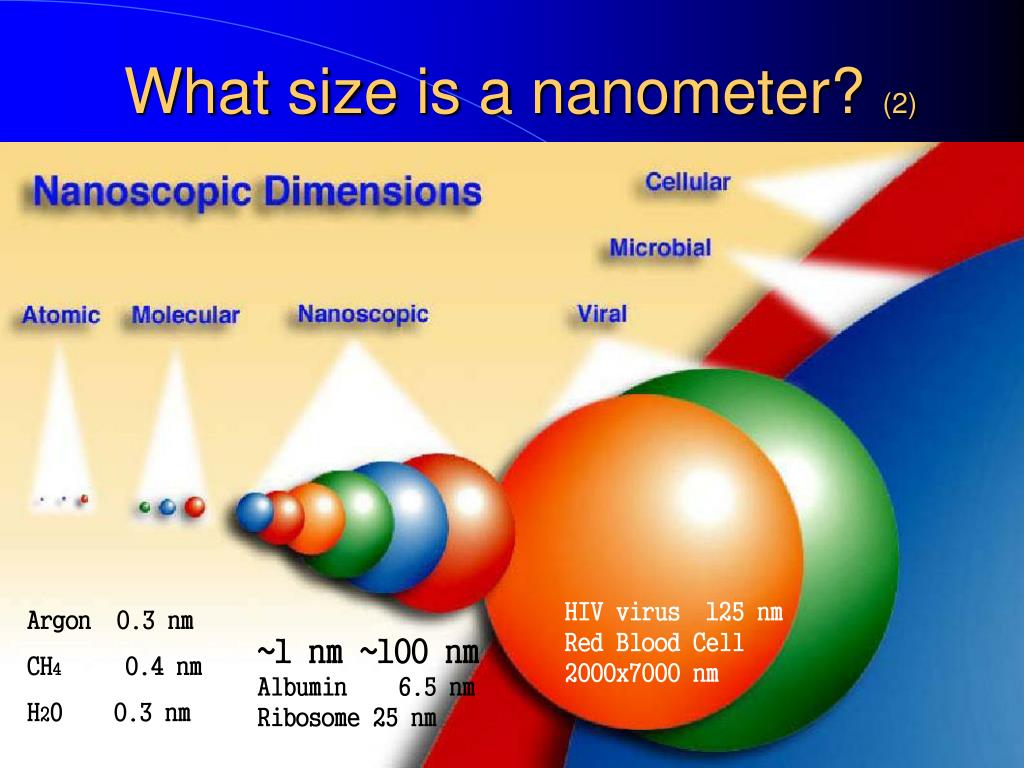The infographic titled "What Size is a Nanometer?" showcases a visual representation of various objects and their sizes within the nanometer scale. The title is prominently displayed in bright orange letters at the top against a blue background, followed by the term "nanoscopic dimensions." The infographic categorizes objects with spotlighted sections labeled: atomic, molecular, nanoscopic, viral, microbial, and cellular. Each section contains colored circles or spheres (blue, red, orange, green) indicating different objects and their corresponding sizes in nanometers.

In the atomic section, argon is shown at 0.3 nanometers, CH4 (methane) at 0.4 nanometers, and H2O (water) at 0.3 nanometers. Moving to the nanoscopic category, albumin is listed at 6.5 nanometers and ribosomes at 25 nanometers. The viral section features the HIV virus at 125 nanometers. The microbial category includes the red blood cell, which measures 2,000 by 7,000 nanometers, making it the largest in the series. Each size is meticulously detailed, providing a comprehensive understanding of the scale of various particles and organisms.